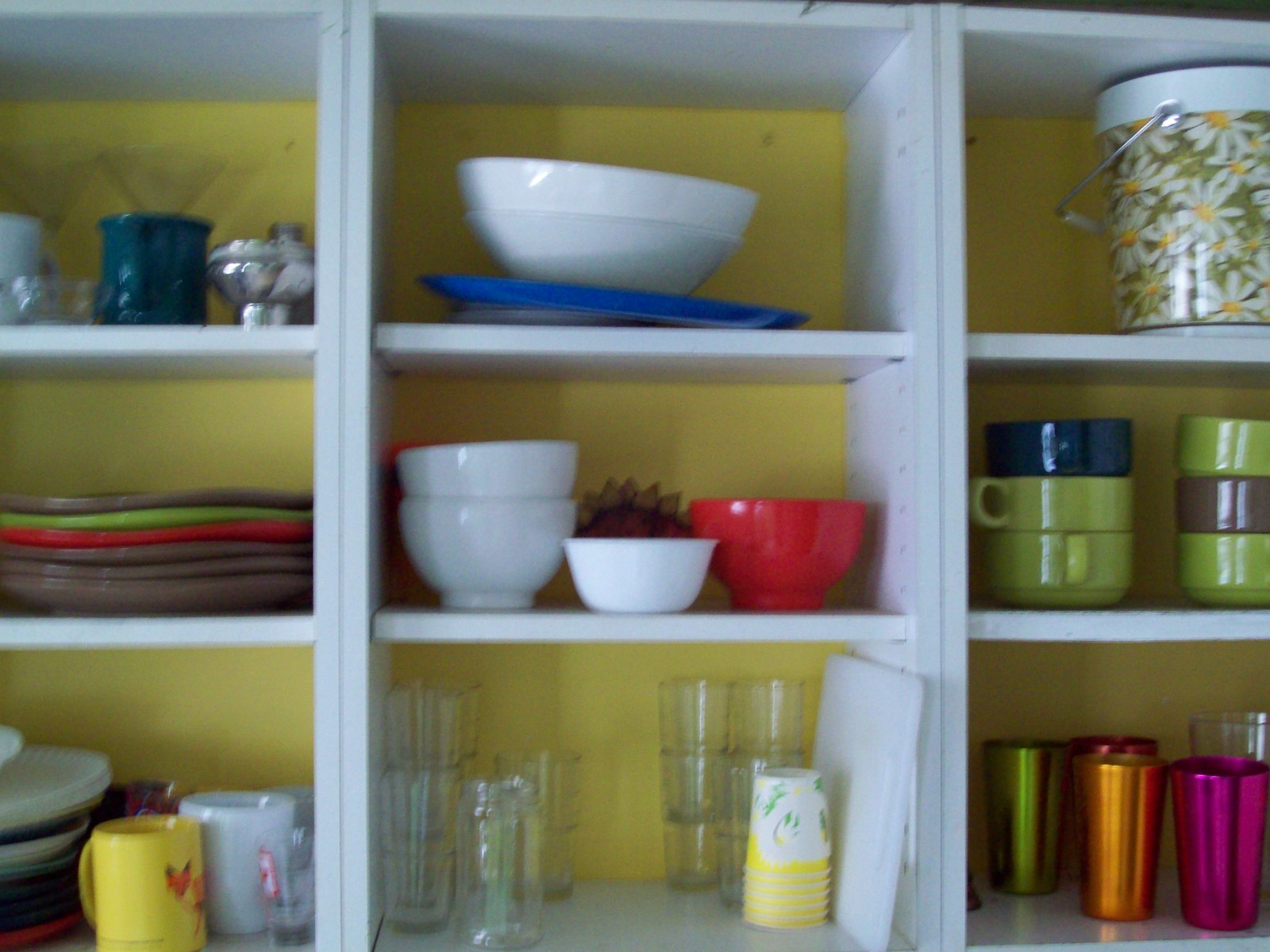The image showcases a section of kitchen cabinet shelving against a yellow wall, featuring white cabinets divided into individual cubby spaces. Each cubby contains a variety of kitchenware:

- **Top Left Cubby**: Contains a collection of mugs, including one white and one navy mug, alongside a silver object.
- **Below Top Left Cubby**: Filled with plates in diverse colors—brown, red, and green.
- **Below the Plate Cubby**: Houses additional dishes, including a yellow mug and a white glass.
- **Top Middle Cubby**: Displays a large white bowl resting on top of a blue plate.
- **Middle Middle Cubby**: Contains two white bowls stacked together, a single white bowl, and a red bowl next to it.
- **Bottom Middle Cubby**: Stores an assortment of glass cups stacked together, accompanied by a white cutting board and stacked yellow cups.
- **Top Right Cubby**: Features a decorative canister with floral designs.
- **Below Top Right Cubby**: Holds blue and green mugs stacked together.
- **Bottom Right Cubby**: Contains taller cups standing in a row, displaying metallic finishes in pink, orange, and green.

Each item is meticulously placed, contributing to an organized, colorful, and visually engaging kitchen display.